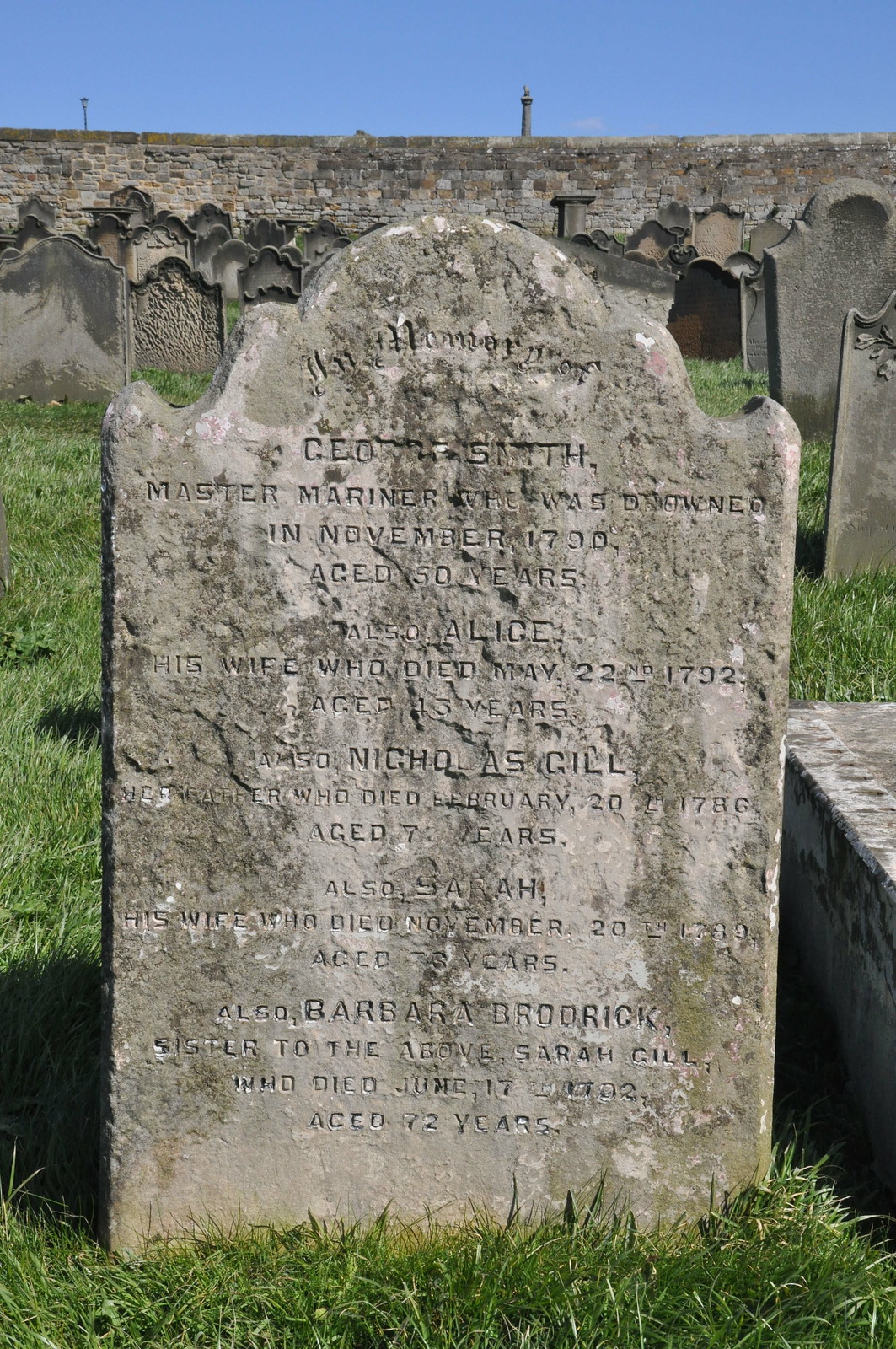The image captures a close-up of a very worn gravestone in an old graveyard. The gravestone itself is a vertical rectangle with rounded scalloped edges at the top, filled with over ten lines of engraved capital letters, many of which are difficult to read due to age and wear. The stone looks aged, with varying colors marking its surface. The legible parts of the inscription mention "Smith," possibly Cedric Smith, a Master Mariner who drowned in November 1790 at the age of 50. It also mentions his wife, Alice, who died on May 22, 1792, aged 45. Another name, Nicholas Gill, who died on January 20, 1786, aged 77, appears alongside Sarah Gill, who possibly died in November 1790 at the age of 70 or 73. Barbara Broderick, sister to Sarah Gill, is also inscribed, having died on June 17 at 72 years old. In the background, rows of similar gravestones stretch out to the horizon under a sliver of clear, bright blue sky. Green grass surrounds the graves, particularly noticeable in front and to the left of the pictured gravestone. A stone wall composed of variously colored stones marks the border of the graveyard, with a hint of a platform visible to the right of the gravestone.